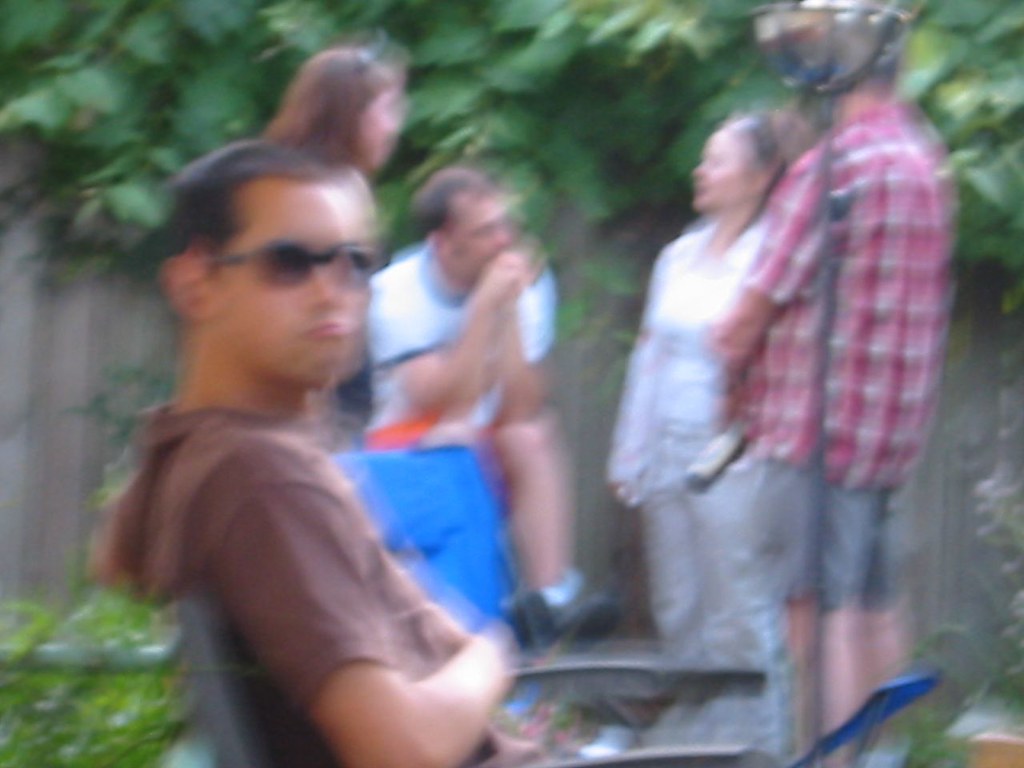A blurry photograph captures a lively backyard scene on a sunny summer day. In the foreground, a young man with brown hair and wearing sunglasses sits with a laptop on his lap. He is dressed in a brown, short-sleeved hooded t-shirt and is making a funny, exaggerated frown at the camera. Behind him, running along the edge of the yard, there's a fence adorned with lush greenery and perhaps vines cascading over the top. In the background, partially obscured by the blur, four people are gathered in a semi-circle engaged in conversation. Three of them are standing while one appears to be seated on what might be a picnic table. The group seems relaxed and enjoying each other's company in the warm outdoor setting.